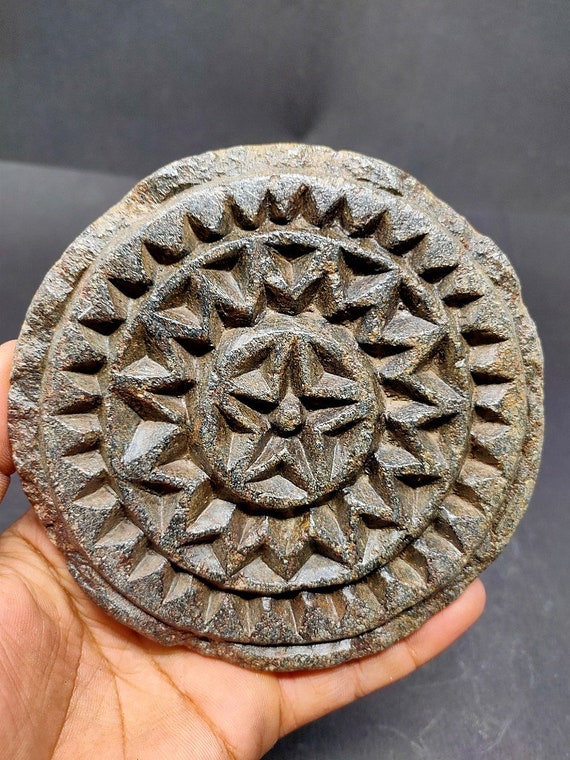In the vertically oriented, realistic photograph with a gray, indistinct background, we see a person's hand occupying the bottom left quadrant of the image, palm-side up, with their pinky finger and part of their thumb visible. The hand extends roughly halfway into the picture. In the center of the hand, there is a large, circular disc, approximately six to eight inches in diameter, which seems to be made of a stone-like material. The disc features a detailed, intricate design, with a central star surrounded by multiple concentric circles, each containing additional star patterns with numerous points. The design is deeply engraved, giving it a three-dimensional appearance. The main focus of the image is the hand holding this ornate, possibly archaeological artifact or artistic piece.